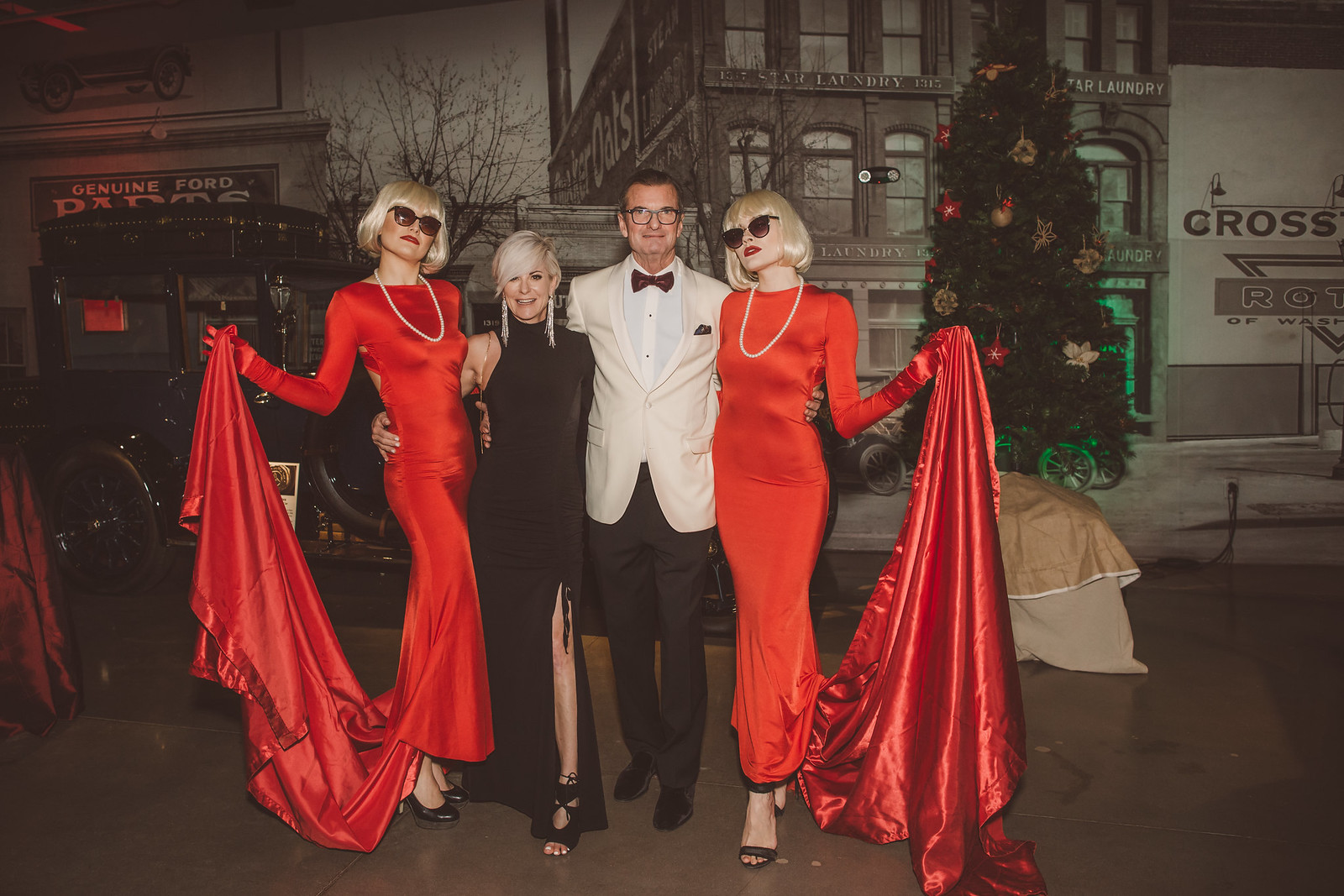In this detailed, color, landscape-oriented photograph, four individuals stand together in the center, facing the viewer, with their arms around each other. The man in the middle sports a white tuxedo jacket, black bow tie, black pants, black shoes, and wire-rim glasses. To his left is a woman in a long black dress that shows some leg, adorned with duster earrings, and blonde hair. She has her right arm around the waist of another woman. The second woman, to the man's right, also wears a long black dress, exposing her shoulders, and has diamond-like long earrings. Flanking the group, on both sides, are two identically dressed women in striking red satin gowns with gloves, holding up the trains of their dresses. These two women, also wearing blonde wigs, dark sunglasses, and white pearl necklaces, create a symmetrical visual effect.

In the background, there is a decorated Christmas tree with a gold blanket underneath, suggesting a festive setting. The backdrop features a city mural depicting strip mall locations, including signage for "Genuine Ford Parts," and old apartment buildings, evoking a 1930s feel. An old Model T car adds to the vintage ambiance. They stand on wood plank flooring, and the photograph captures the scene with a style of photographic representational realism.